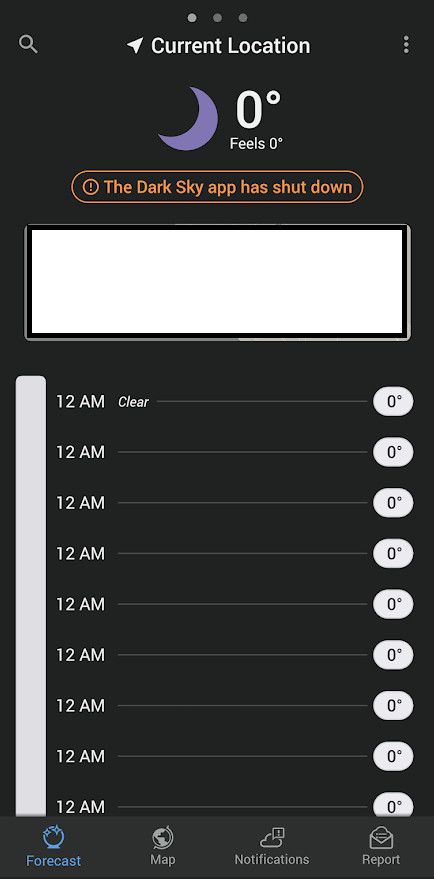A gray-toned weather app interface displays the current location and the forecast for "Blue Moon." The temperature is noted as 0 degrees and it feels like 0 degrees. An orange oval indicates an advisory, stating, "Expect the dark sky to push it down." In white text, it highlights that at 12 a.m., the weather will be clear with 0 degrees.

Repeatedly, the hours following and including 12 a.m. are shown, all with a forecast of clear skies and a temperature of 0 degrees. A blue text bar below suggests options such as "Forecast," "Map," "Cloud," "Notifications," and an envelope icon labeled "Report."

Overall, the interface presents a minimalist and sleek layout with multiple elements arranged in lines, providing various weather details and functionalities.